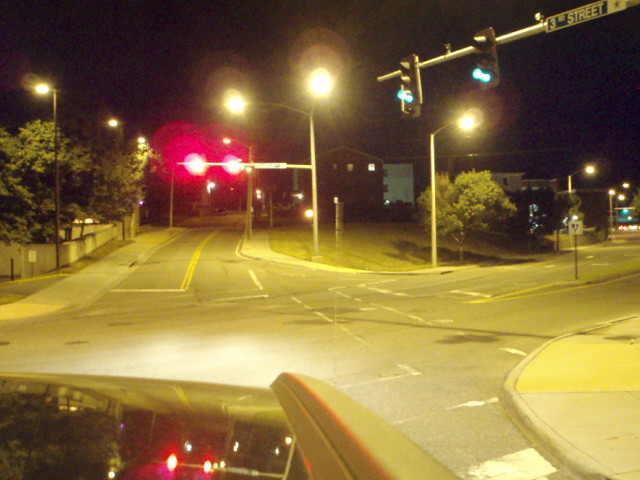A nighttime photograph taken from the inside of a car at a four-way intersection. The image is viewed through the windshield, revealing the car's hood below, which reflects the surrounding streetlights and traffic signals. The scene is framed by the red light visible for the photographer's direction, while the green light for the crossing traffic illuminates the area. Each direction of the intersection contains a single lane of traffic. In the background, residential buildings such as apartments or condos are partially visible against the night sky. Trees and patches of grass line the opposite side of the street, with clearly marked pedestrian crossings hinting at a well-structured urban setting.